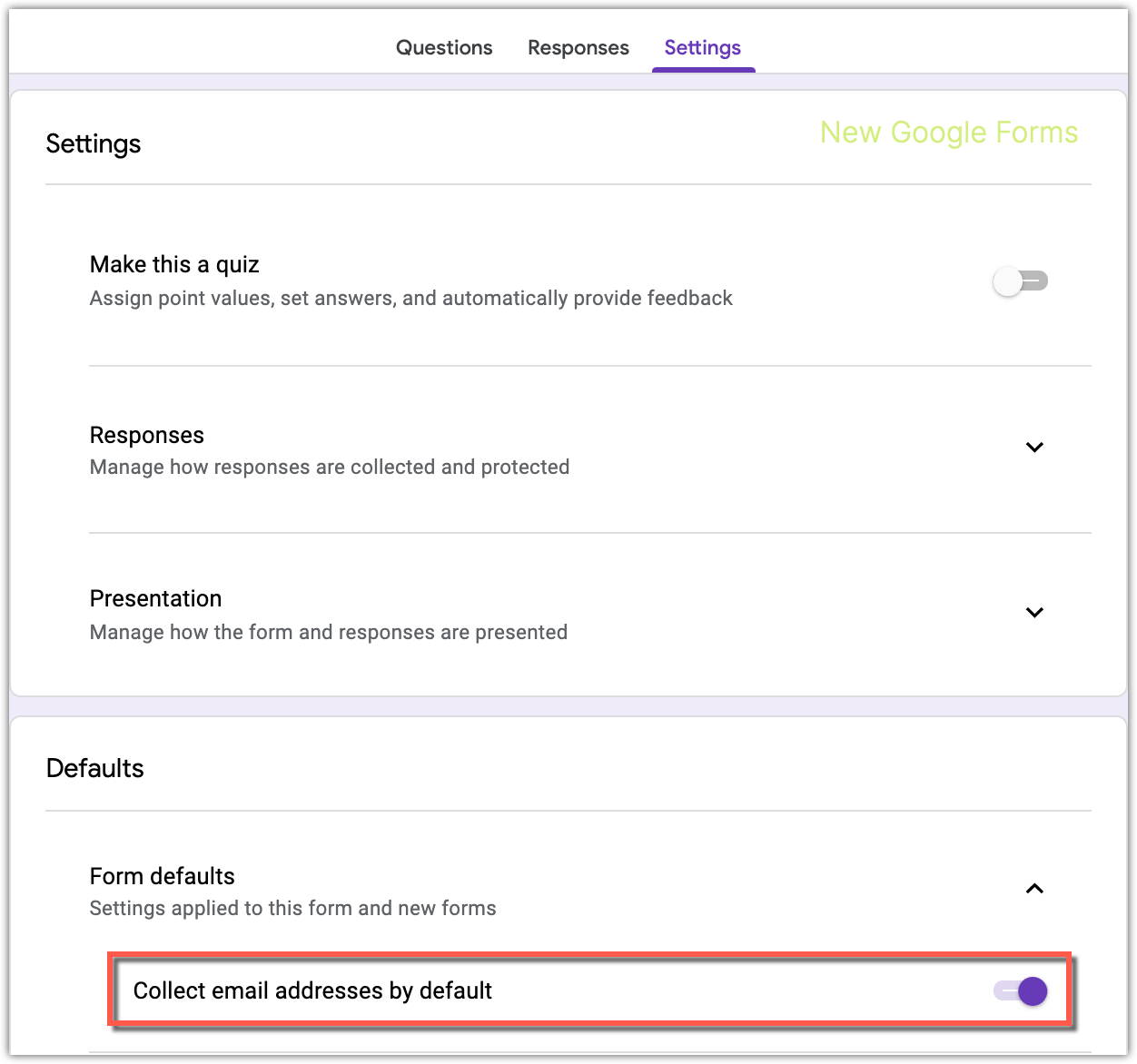This is a detailed descriptive caption for the image:

The screenshot captures the settings page of a website, identified as the settings tab by the highlighted word "Settings" in purple, underlined with a matching purple line. At the top of the page, there are three tabs: "Questions," "Responses," and "Settings," with the current focus on the "Settings" tab. The header of the page prominently displays the word "Settings," with "New Google Forms" written in green text on the right side.

Beneath the header, there are several sections with various options, starting with "Make this a quiz," which includes the ability to assign point values, set answers, and automatically provide feedback. This option features a toggle button on the right, currently in the off position.

Following that, the "Responses" section allows users to manage how responses are collected and protected, and the "Presentation" section manages how the form and responses are presented. Both of these sections include downward-pointing arrows indicating they can be expanded for more options.

The final section, titled "Defaults," contains "Form Defaults" settings, which apply both to the current form and new forms. This section has been expanded, indicated by an upward-pointing arrow. One specific option, "Collect email addresses by default," is toggled on, with the toggle button displayed in purple. Notably, a red rectangular outline has been added around this option, emphasizing it as a key feature included via editing.